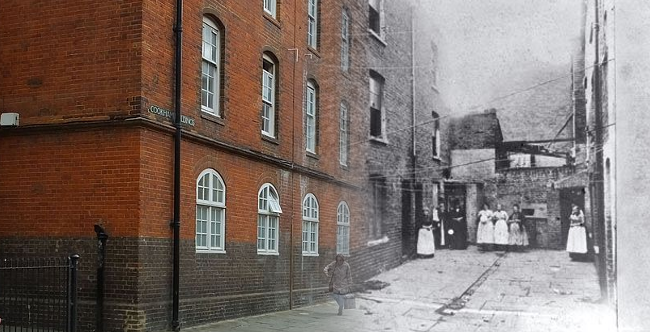This image is a composite of two different photographs creating a seamless transition between the past and present of a historical site. On the left, we see the present-day depiction of a giant red brick building with distinct windows featuring unique frames and arch designs. A woman in modern attire walks partially in color, adding a touch of vibrancy to this side of the image. As we move to the right, the image fades into a black and white photograph, likely dating back over a hundred years. This side captures the same building in its earlier state, complete with a group of people in period clothing – white dresses and suits – posing near a garage. The black and white portion is noticeably more faded, capturing the passage of time. The building's architectural details, including its red bricks and brown base, remain consistent across both halves, offering a striking contrast between the lively present and the nostalgic past.